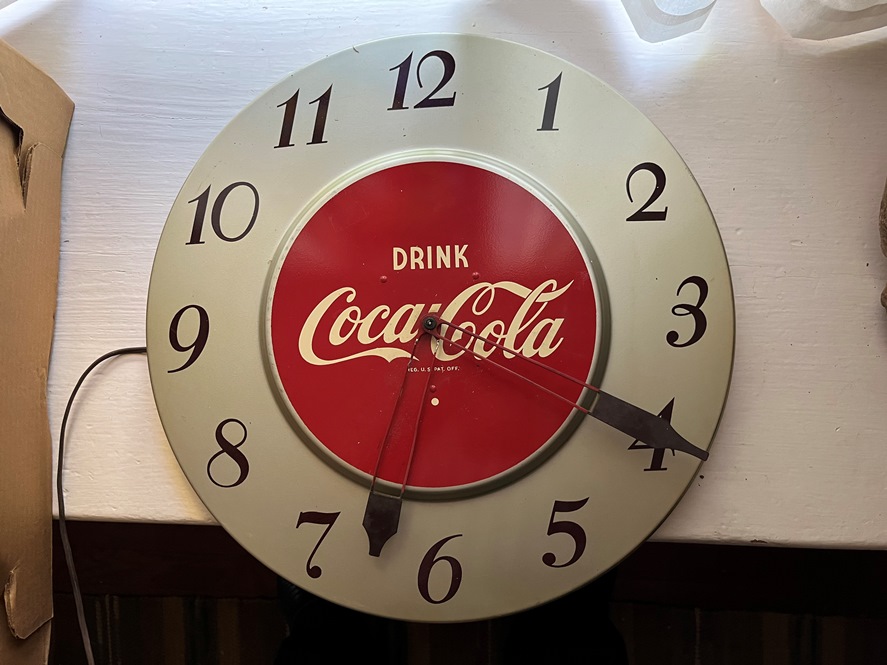This photograph features a close-up of a Coca-Cola wall clock, which is uniquely oriented 90 degrees, placing the top (12 o'clock) on the right-hand side of the image. The clock has a gray outer casing with black analog numbers. The black minute hand is at the "4" and the black hour hand is positioned between the "6" and "7," indicating the current time as 6:20. At the center of the clock is a raised red circle, prominently displaying the iconic "Drink Coca-Cola" logo in white letters. A red wire and a cord can be seen extending from the clock's center towards the "9" on the clock face (top of the image). 

The clock is resting on a white tablecloth which covers a surface flanked by a cardboard box on the left. A white curtain is partially visible towards the upper right of the frame, while a dark background and floor are obscured by shadow. Light cascades into the image from the top, highlighting the setup.